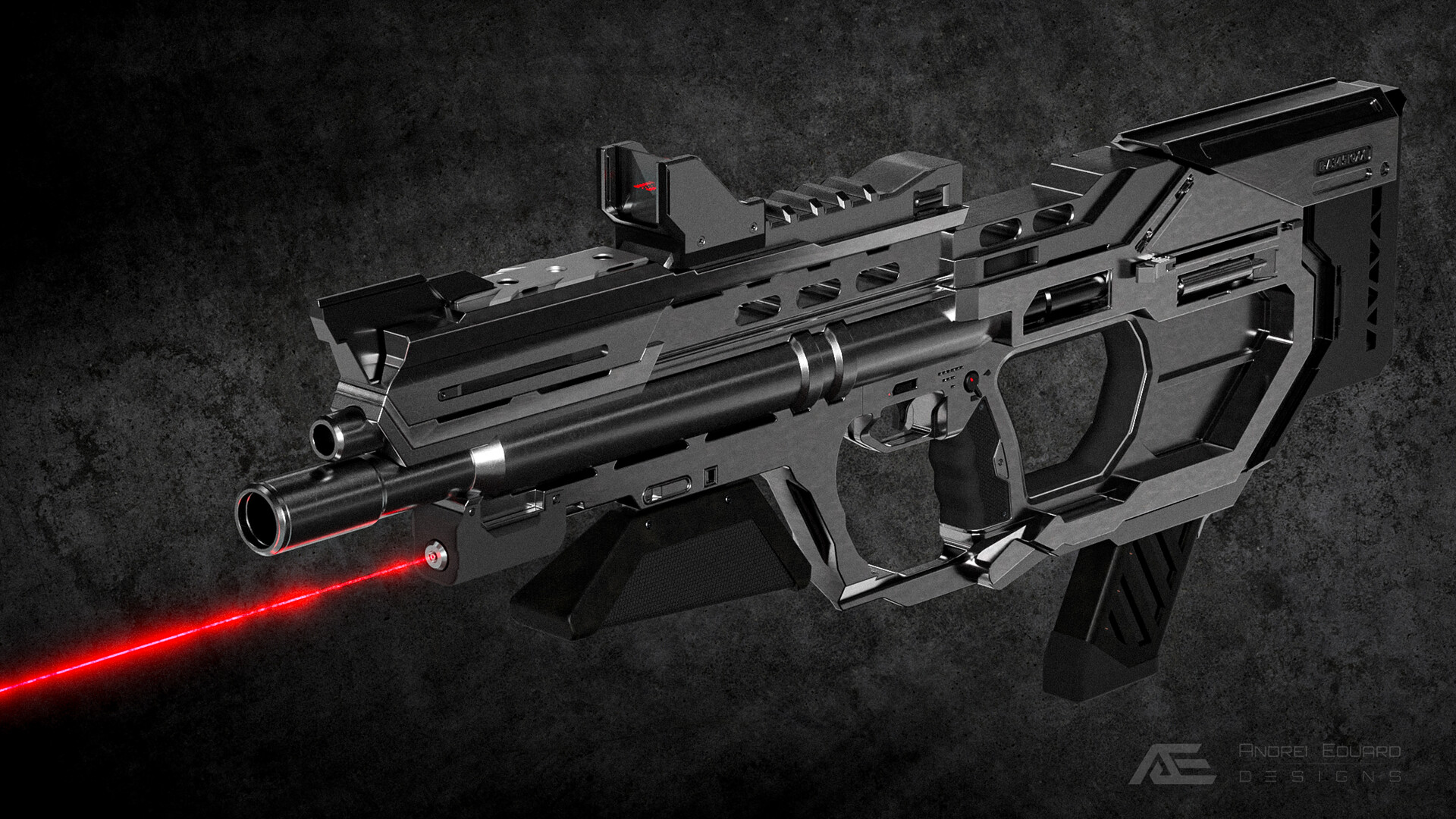In this detailed rectangular image, we see a black and gray marbleized background featuring a sleek, black machine gun pointing to the left. The gun, crafted by Andre Edouard Designs, as denoted by the "A.E." logo in the bottom right corner, appears to be made of shiny black metal. Notable details include a horizontally positioned cylinder near the top, possibly indicating the barrel, although it doesn't protrude significantly. The gun has a large handle extending from the top to the bottom and a red laser beam emanating from the front bottom, providing a stark contrast to the grayscale surroundings. Additionally, an eye sight with a red light is positioned atop the gun, possibly serving as a guidance system, further highlighting its precision and functionality. The image is dominated by its monochromatic tones, accentuating the futuristic and sophisticated design of the weapon.